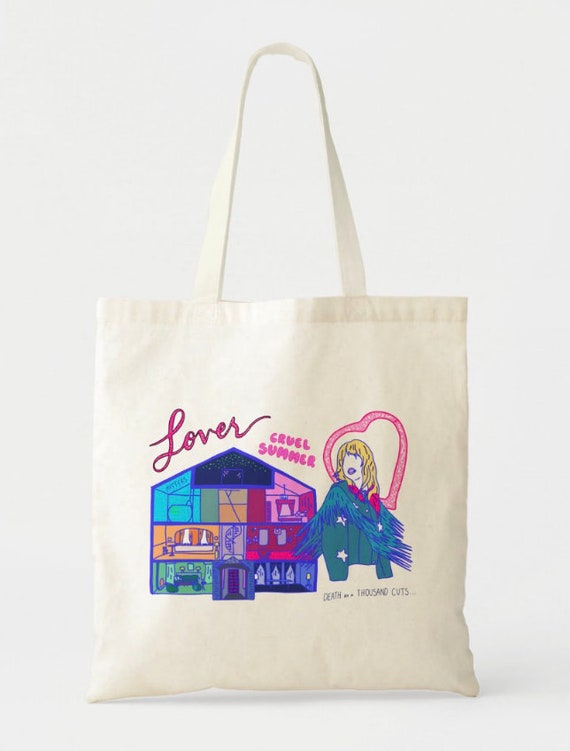The photograph depicts a white canvas tote bag with a long strap, set against a white background, lending a clear and distraction-free view. The tote bag features pink cursive lettering that reads "Lover" and puffy print text stating "Cruel Summer." The bag is primarily white with an eggshell hue. Central to the design is an illustration of a cutaway, dollhouse-like suburban home where every room is vividly colored—blue, pink, orange, green, and more. Stairs connect the rooms, creating a multi-story visual effect. Adjacent to this vibrant house is an intriguing female figure with blonde hair, a red mouth, and apparently no eyes. The figure's unconventional design includes what looks like a head floating above a body-less sweater adorned with a scarf made of bird feathers. A heart shape encircles her head, completing the whimsical and detailed artwork on the bag.